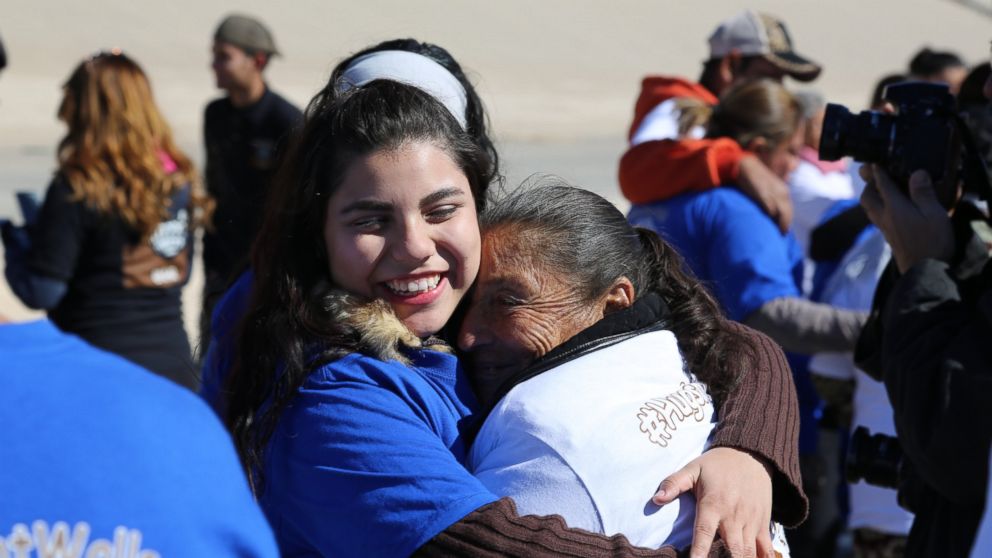The outdoor, candid photograph captures a heartwarming scene of intergenerational care and compassion. In the center, a young woman with black hair, wearing a blue short-sleeve shirt over a brown sweater and a white headband, embraces an older woman who appears to be Hispanic, dressed in a white jacket with the hashtag "hugs" printed on it. Both women are smiling, with the younger woman's eyes closed, radiating warmth and affection. 

Surrounding this pair are several other people, predominantly dressed in blue t-shirts, likely indicative of a volunteer group or mission. These helpers, some of whom are seen comforting and embracing older individuals not in uniform, create an atmosphere of nurturing support. A noticeable man in the background, wearing a gray baseball cap and a red and white jacket, also participates in the communal embrace, suggesting possible leadership or coordination among the volunteers.

Amidst this backdrop, there are glimpses of other figures: a woman in a brown jacket with red hair, turning away from the camera, and a man wearing a gray cap, visible in profile. Despite the slightly blurred or out-of-focus areas, the collective image vividly conveys a powerful sense of solidarity, care, and community spirit.